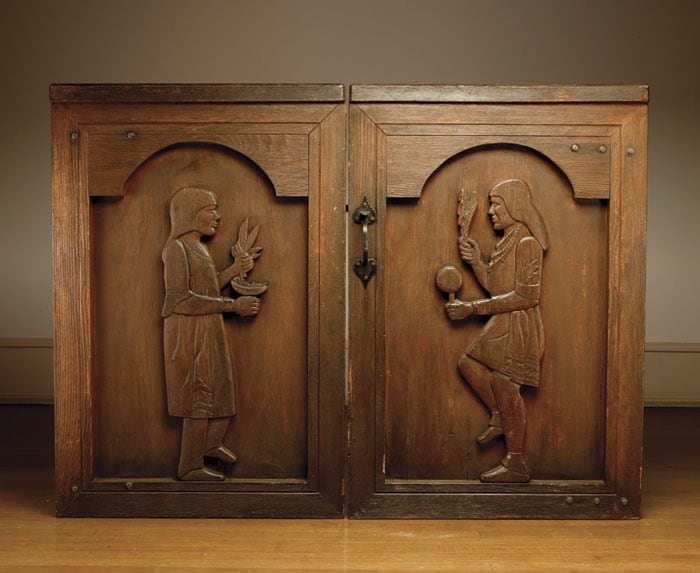The image features a single, ornate wooden cabinet with dual doors, each adorned with a meticulous engraving. The overall hue of the cabinet is a deep brown. One door presents the detailed profile of a villager or Native American figure, facing inward, and holding what appears to be corn or possibly ceremonial objects, suggesting a ritualistic scene. The other door mirrors the detailed craftsmanship, showcasing a figure that evokes a Roman persona holding a chalice in one hand and a pot in the other, also facing inward. The cabinet is crowned with a curved top, enhancing its antique appearance. Despite the cabinet having two doors, it is equipped with just one handle. The engravings on each door make the cabinet resemble two side-by-side nightstands, but they are part of a single piece, embodying an old-world charm and rich cultural narrative.